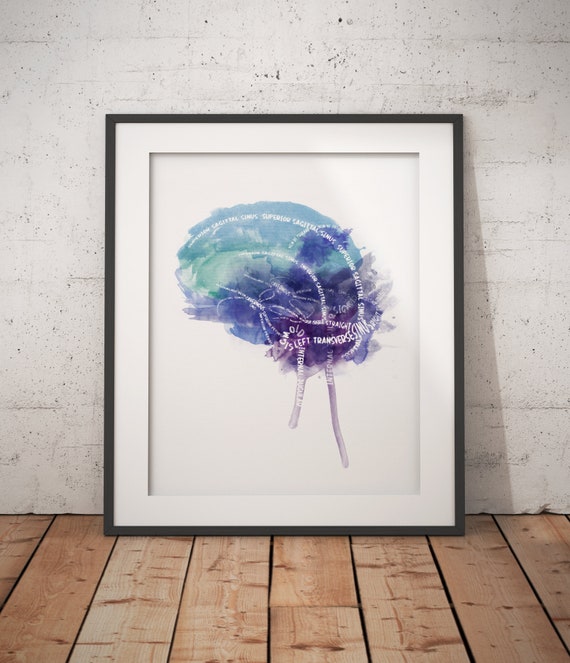The photograph captures a detailed scene of a framed painting positioned on a brown wooden floor in an indoor setting, leaning against a white brick wall. The frame itself is black with an inner matte white border, enclosing a painting with a white background. Central to this painting is a brain-like shape, vividly rendered in a watercolor style with an array of colors including blue, turquoise, teal, purple, and pink. This brain shape is intricately overlaid with very small white text, featuring motivational or inspirational words that are spaced throughout the colored area. Despite the clarity of the overall image, the text is challenging to read due to its size. Natural indoor lighting highlights the vibrant colors and details of both the painting and its setting.